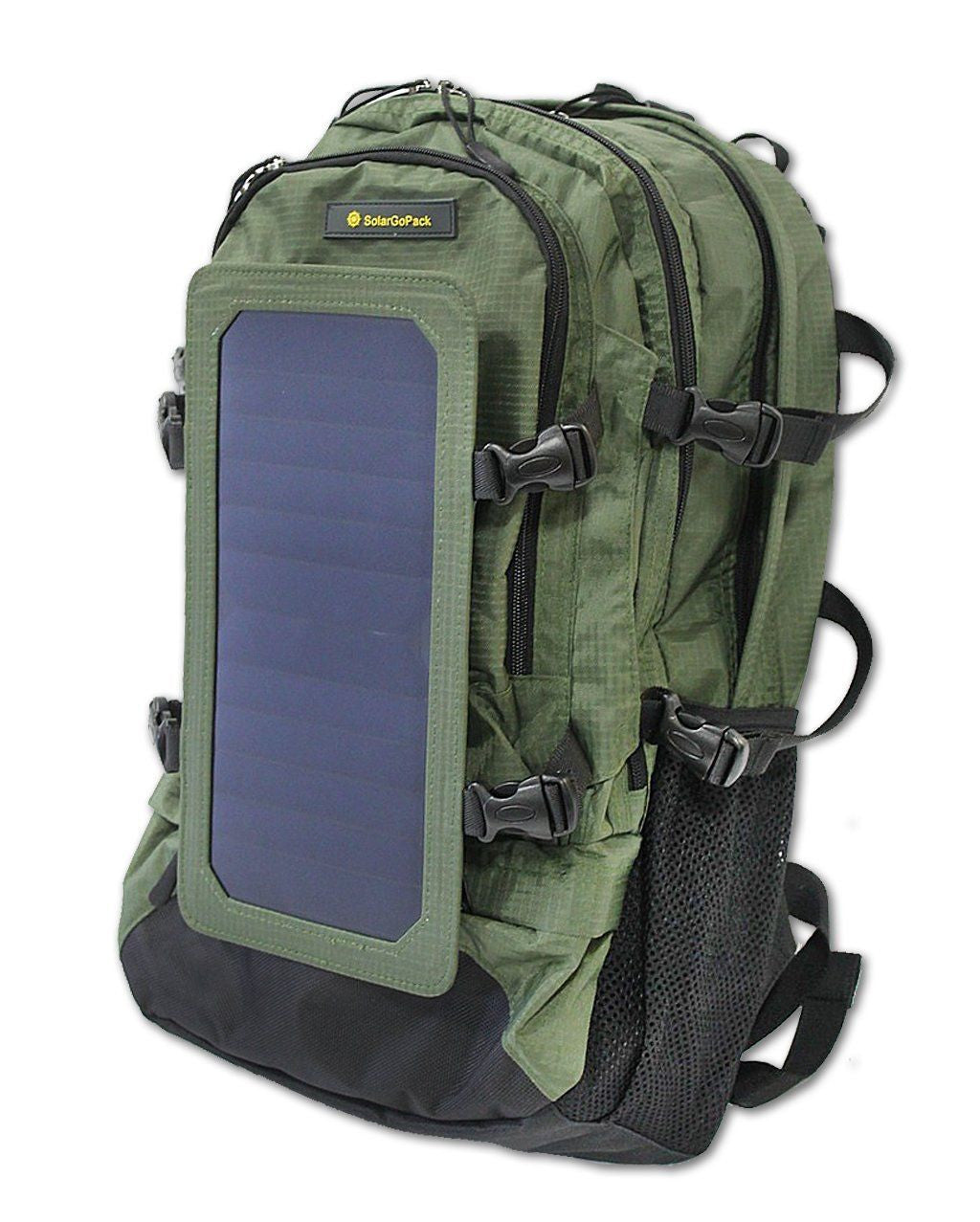This image features a high-quality green backpack designed for camping or hiking, prominently displayed on a transparent background. The backpack, labeled "Solar Go Pack" in yellow text, includes a solar panel which seems integrated into a rectangular section at the back, suggesting that it can be used to power electronic devices on the go. It has three sizable zippered compartments with black zippers and clips, along with two side mesh pouches located on the lower half, ideal for holding drinks. Additional straps and belt-like clips secure the backpack's structure, ensuring it can carry a significant load comfortably. The front of the backpack is blue framed by green, with black accents completing its rugged look.